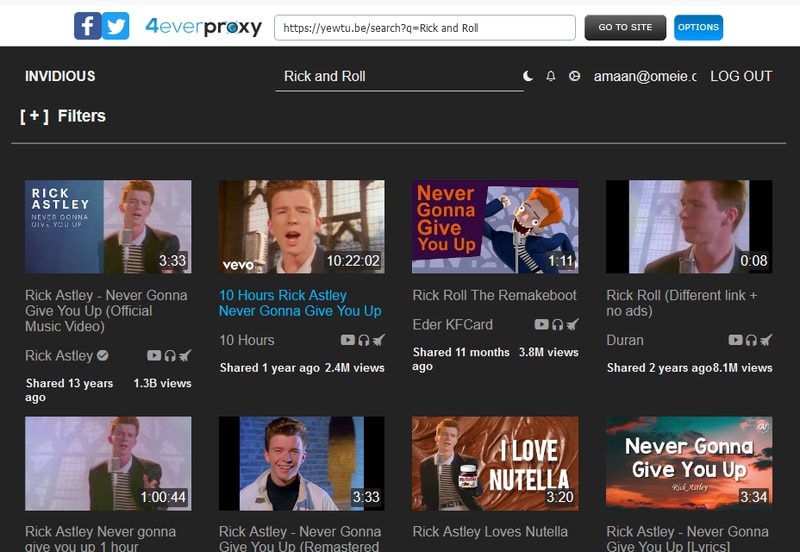The image depicts a web page with a predominantly white upper section transitioning to a black background beneath. 

At the top, two recognizable social media icons are displayed—a blue square with a white "F" representing Facebook, and a lighter blue square with a white bird, signifying Twitter. Below these icons, the word "forever" appears in blue text, with "proxy" next to it in black. 

Centered on the page is a white rectangular field containing "https.com" and beside it, a black rectangle with "go to site" in white text. Adjacent, a blue rectangle with "options" in white text is visible.

Further down, the background of the page turns black with the word "NVIDIA" prominently displayed in white. Below this, a line reads "Rick and Roll" and is accompanied by three symbols: a white crescent, a white bell, and a white circle. The text "a-n-a-a-n-a-t-o-n-e-i-e dot" appears beneath these symbols, followed by the word "logout."

Continuing down, a white plus sign in brackets followed by the word "filters" in white text is shown. This section is divided by a thin white line.

The lower part of the image is populated by four video thumbnails organized in rows. The first row of videos includes:
1. "Rick Astley - Never Gonna Give You Up (Official Music Video)"
2. "Ten Hours of Rick Astley - Never Gonna Give You Up"
3. "Rick Roll [Remake Bo]"
4. "Rick Roll (Differently) [No Ads]"

The second row of videos features:
1. "Never Gonna Give You Up - One Hour"
2. "Never Gonna Give You Up - Be Mastik"
3. "Rick Astley - Love Nutella"
4. "Rick Astley - Love (Never Gonna Give You Up) [Lyrics]"